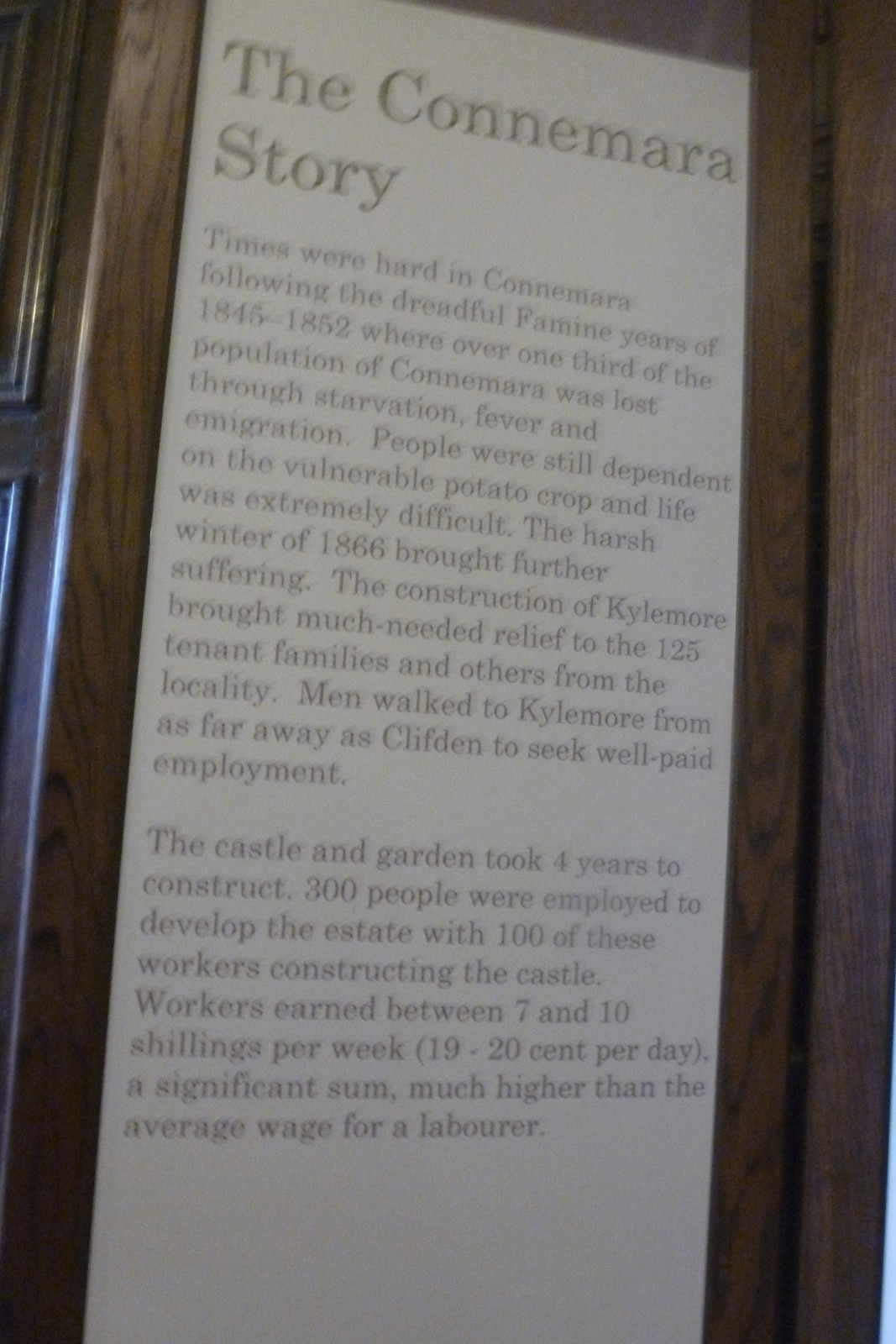The image features a framed display in a museum, showcasing a large white board titled "The Connemara Story" in prominent letters. The board contains two paragraphs of text that recount the hardships faced by the people of Connemara during and after the Irish potato famine from 1845 to 1852, which resulted in the loss of over one-third of the population due to starvation, fever, and emigration. The text describes the continued reliance on the fragile potato crop and the extreme difficulties experienced during this period. It also highlights the additional suffering caused by the harsh winter of 1866 and mentions the construction of Calamar, which provided much-needed relief and employment to 125 tenant families and others from the local area. Men traveled from as far away as Clifton to find well-paid jobs. The photograph appears slightly blurred, suggesting it was taken while the person was moving.